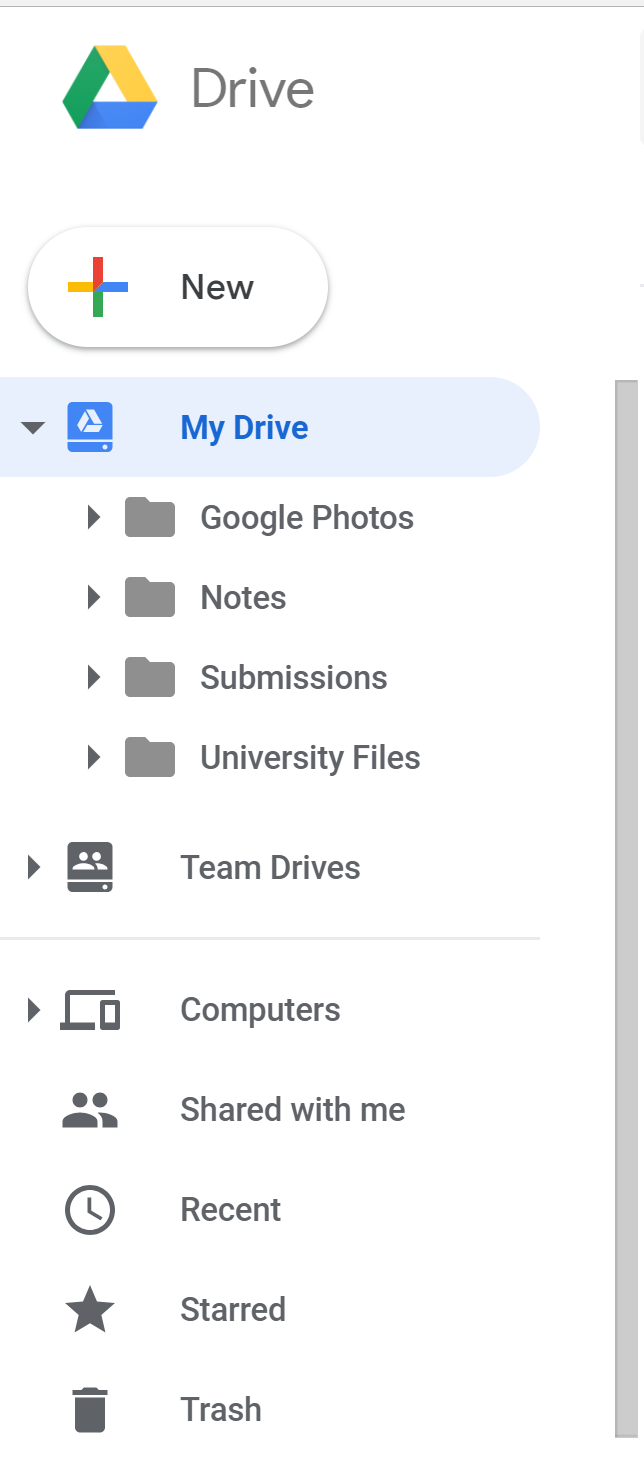The image depicts a Google Drive interface. At the top, there is the iconic Google Drive logo featuring four colors: red at the top, yellow to the left, blue to the right, and green below, all surrounding a central plus sign. This indicates the option to add new items. The interface shows various folders created by the instructor for their "My Drive," which includes sections like Google Photos, Notes, Submissions, and University Files. Below these, there are additional folders labeled as Steam Drives, symbolizing some external or additional drives. There are icons representing shared items (two people icon), recent files (clock icon), starred items (star icon), and trash (trash bin icon), all located on the left side of the interface. A gray vertical bar on the right side acts as a separator for different sections within the Google Drive. The overall display shows various folders and filter options available in Google Drive.